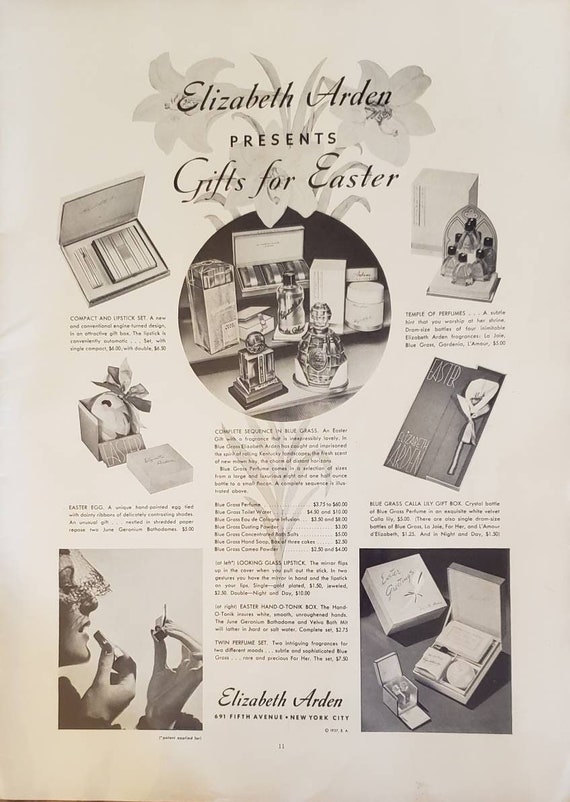This black and white magazine advertisement from the 1940s or 1950s features an Easter-themed display of gifts by Elizabeth Arden, a renowned name in beauty and style, known for her store on Fifth Avenue in New York City. The title prominently states, "Elizabeth Arden Presents Gifts for Easter," accompanied by a variety of suggested presents aimed at women. Notably, the ad showcases a compact and lipstick set, a perfume temple, a Blue Grass collection, and a Calla Lily gift box, among other elegant items. On the left side, there is what appears to be a cigarette case or a makeup compact. At the center, a round vignette highlights perfume bottles displayed on a stand. To the right, there is a collection of perfume bottles, sachets, and Easter cards, as well as a small box with an open bottle. The background includes floral motifs, enhancing the festive theme. At the bottom left of the ad, a woman in a half veil is depicted, gracefully applying lipstick while holding a compact. On the bottom right, there is a gift set and another open box of beauty products, possibly featuring a diary with a pen shaped like a flower. The advertisement contains text descriptions and pricing information for the various items, although the specific text is too small to read.